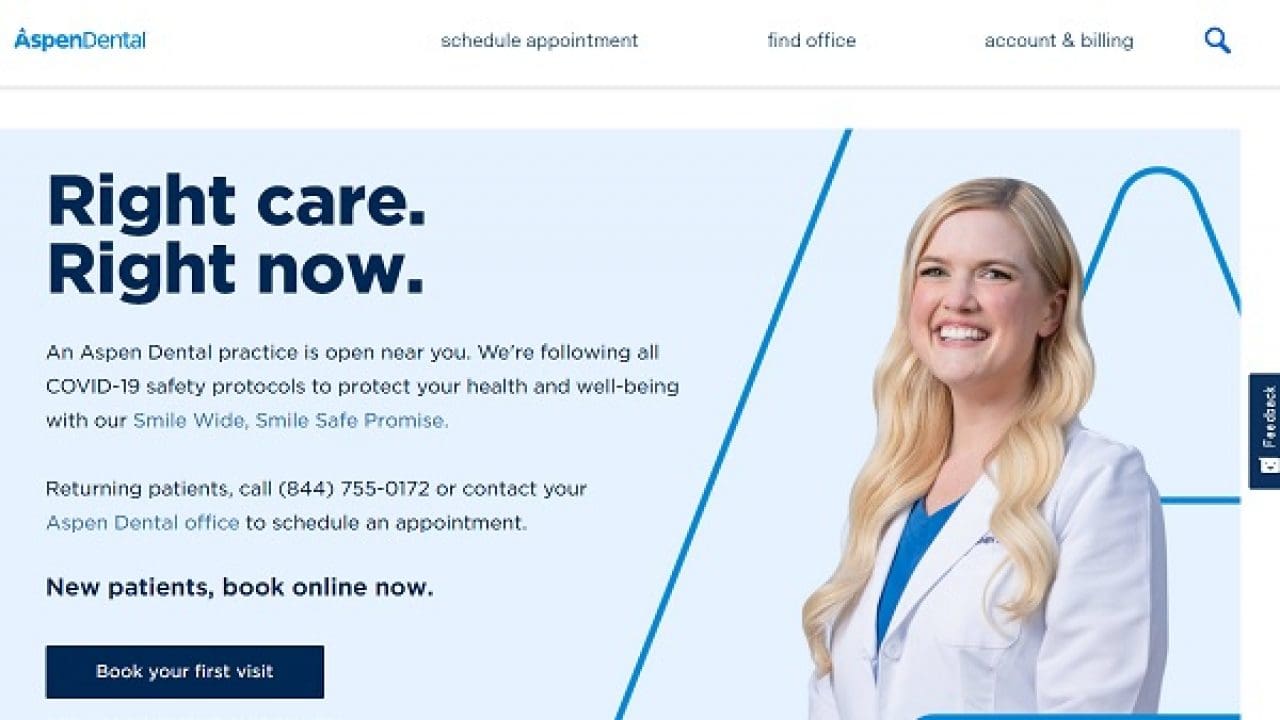The image features a webpage for Aspen Dental set against a white background. In the upper left corner, the Aspen Dental logo is displayed in blue text, adjacent to a navigation bar with dark blue text that reads "Schedule Appointment," "Find Office," and "Account and Billing." In the upper right corner, there is a blue magnifying glass icon. Below this, a gray horizontal line spans the width of the page.

The next section has a light blue background with dark blue text. In the upper left corner, bold text reads, "Right Care, Right Now." Below this, lighter text informs visitors: "An Aspen Dental practice is open near you. We're following all COVID-19 safety protocols to protect your health and well-being with our smile-wide, smile-safe promise." The following line provides contact information: "Returning patients, call 844-755-0172 or contact your Aspen Dental office to schedule an appointment." Beneath this, bold text encourages new patients: "New Patients, Book Online Now." 

At the bottom, a navy blue rectangle contains white text that says "Book Your Next Visit." To the right, there is an image of a blonde, Caucasian female dentist wearing a lab coat over a V-neck blue t-shirt, smiling warmly.